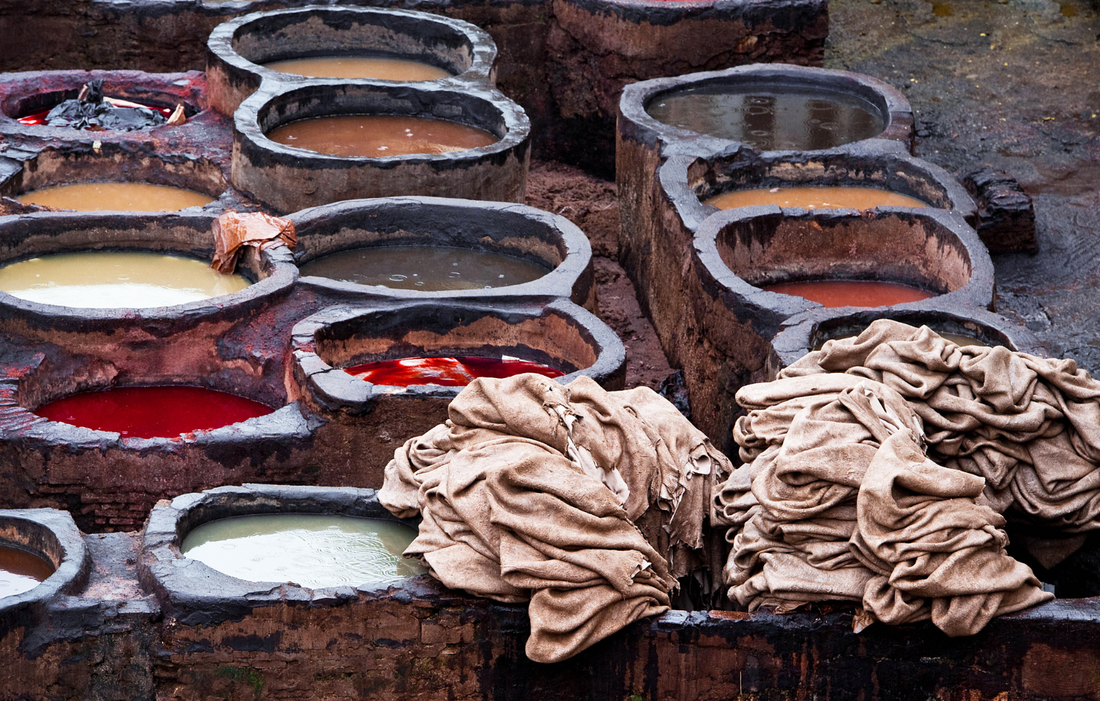The photograph showcases a collection of interconnected, circular containers made of stone or clay, arranged in a square-shaped grid. These vats, filled with various liquids, create a visually striking pattern with colors ranging from light white, off-yellow, shiny red, and blood-red, to murky tan, greenish-brown, and dark brown. The containers, which appear slightly rusted and worn, are covered in a tarp or canvas material in some sections. On the left side of the image, you can see a progression of different colored liquids, starting with a blackish substance at the top, followed by a light orange, a light yellow, and a red liquid, possibly dye. In the foreground, on the bottom right, there is a substantial stack of dirty-looking light brown rags or thin brown cloths, which are damp and overlapping each other. The entire scene exudes a sense of wetness, as if everything in the image is covered in moisture.